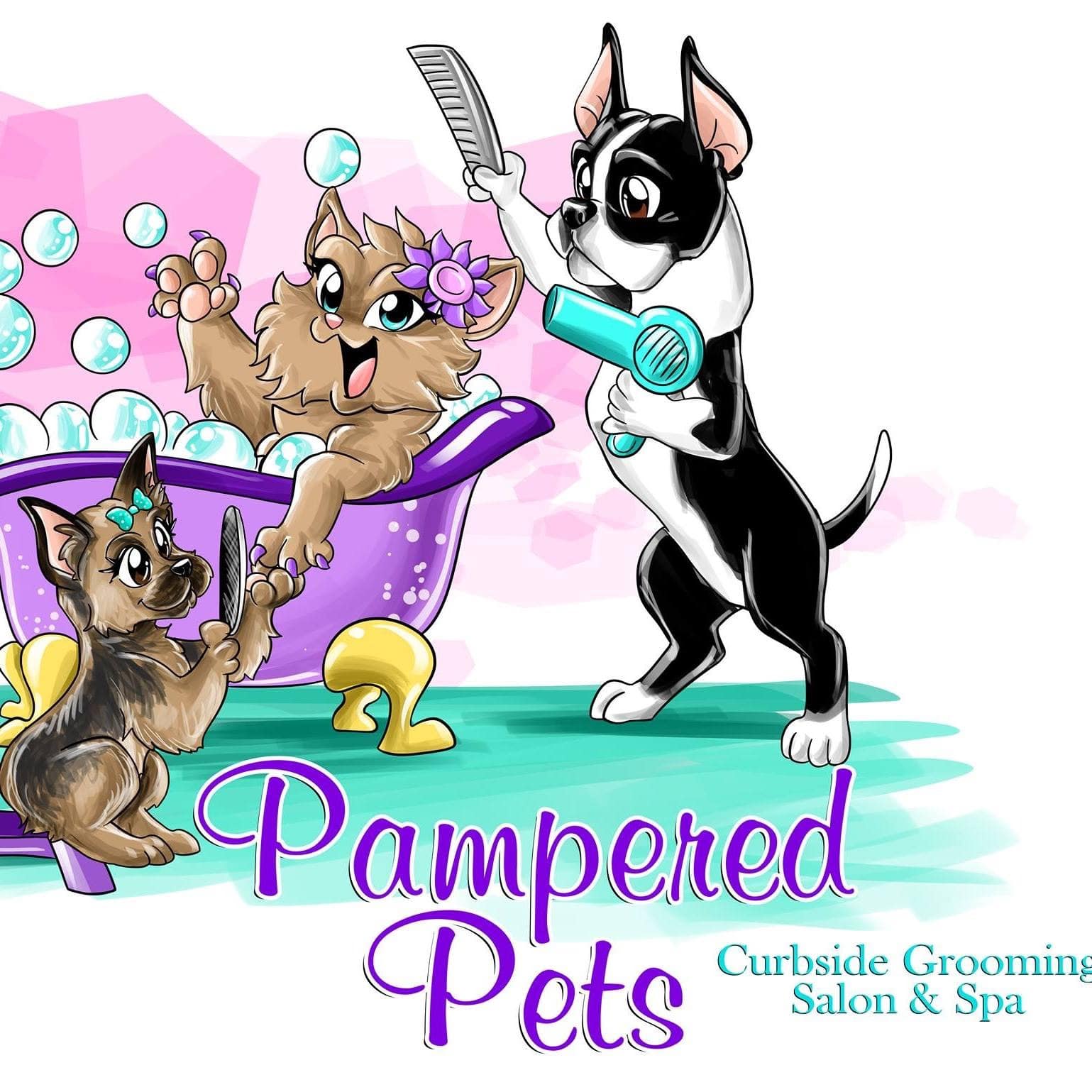This image serves as a vibrant and whimsical advertisement for a company called Pampered Pets, showcasing their curbside grooming salon and spa. Rendered in a charming, cartoony style reminiscent of Japanese anime, the illustration features a light brown cat luxuriating in a bubble bath. The bathtub is a striking purple with elegant gold feet and is filled with light blue bubbles that float in the air around it. The cat, with a contented expression and mouth open in joy, has her right paw extended and her left paw being manicured. Her features include a pink nose, light blue eyes, and a purple flower tucked near her left ear. She sports purple-painted nails, courtesy of a small, diligent brown and black dog who is filing them down. This tiny manicurist wears a teal green bow on its head and sits on a small purple stool.

Flanking the bathtub, another dog—a Boston Terrier with sharp, pointy ears—is busy styling the cat's fur. This black and white dog stands on its hind legs, holding a blue hairdryer in one paw and a metallic silver comb in the other, seemingly focused on delivering top-notch grooming.

Behind this lively scene is a backdrop of hexagonal shapes in varying shades of pink, transitioning from pastel to bubblegum hues. The floor, depicted in teal blue, resembles a blend of marker, scribble, or watercolor techniques, adding to the image's playful ambiance. In the foreground, a prominent purple cursive text reads "Pampered Pets," accompanied by teal blue text declaring "Curbside Grooming Salon and Spa." The overall composition is cheerful and brightly colored, perfect for catching the eye and conveying the delight of a high-end pet pampering service.